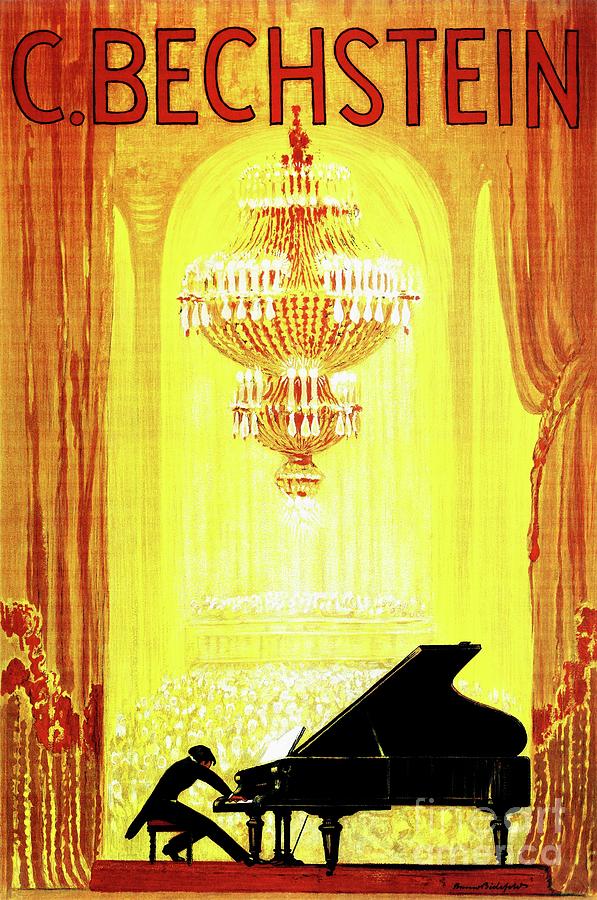The image is a vertically rectangular, multi-color promotional poster, prominently showcasing the name "C. Bechstein" in bold, all-caps red text across the top. It depicts a well-lit, lavish performance stage dominated by warm yellow and red hues. The background is notably yellowish from the stage lights, highlighting the luxurious setting. At the center of the image, a gentleman dressed in a sleek black tuxedo sits on a chair, playing a large black grand piano. Above him hangs a grand, golden chandelier, adding to the opulent atmosphere. Tall orange curtains flank either side of the stage, framing the central figures and drawing attention to the scene. The entire composition emphasizes a dramatic and elegant musical performance, possibly a recital or concert, held in a tastefully adorned venue.